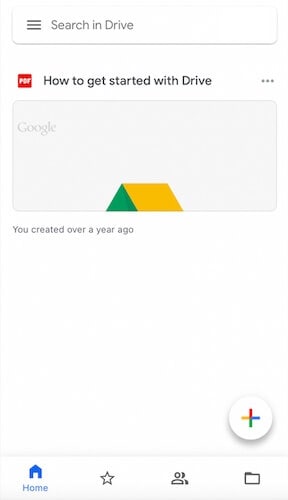A cell phone screenshot depicts a Google Drive interface on a white background. Dominating the top portion of the screen, a red square with white text reads "PDF." Directly beside this, black text states "How to get started with Drive," accompanied by a horizontal array of three dots. Located further up on the left, a gray box contains the word "Google" in similarly gray text. 

Below, a green tent-like icon evokes a classic camping tent with yellow sides, reminiscent of an old-school setup with poles and support strings. Adjacent to this, gray text notes, "You created over a year ago."

The bottom section of the screenshot features the Google Drive toolbar. On the bottom right, there's a circle with Google's multicolored "plus" sign. To the left, highlighted in blue, the "Home" button, marked by a house icon, is prominently displayed. This is followed by a gray star, an icon of two people, and a folder symbol.

The remainder of the screen shows blank white space, completing the interface view.